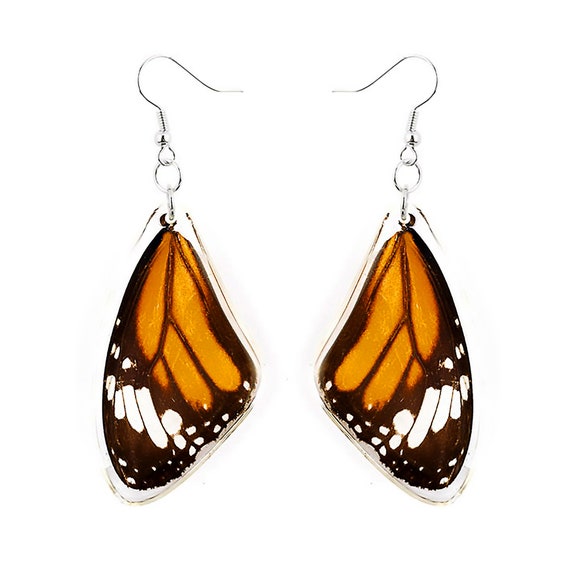This image showcases a pair of intricate, silver hook earrings designed to resemble the wings of a monarch butterfly. Each earring features a simple silver hook at the top, which is threaded through a wire hook attached to a small silver ball. The ball connects to a circular ring, which holds another slightly smaller ring inside it. Hanging from the inner circle is a delicate, life-like representation of a monarch butterfly wing.

The wings, possibly laminated in clear plastic for durability, display the iconic monarch color pattern: a vibrant orange center, interlaced with brown veins, and bordered with a black outline adorned with white dots. This striking combination of colors and delicate features brings an elegant and natural touch to the earrings, making them a captivating accessory that celebrates the beauty of these well-known and distinguished butterflies. Set against a white background, the earrings stand out, showcasing their detailed craftsmanship and vivid colors.